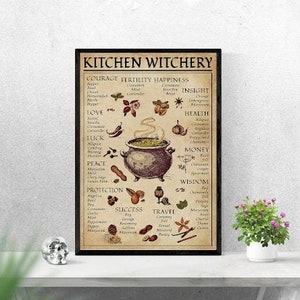This framed artwork features an animated depiction of various kitchen ingredients surrounding a large, dark gray pot at the center. At the top of the frame, the words "Kitchen Witchery" are prominently displayed in black text, underlined by a thin black line. Below this title, a list of different ingredients is rendered in assorted typography. The central pot is filled with green ingredients, emitting whimsical green steam. The background of the artwork is a light brown hue, contrasting with the black square frame that encloses it. The frame is positioned on a white shelf, adorned with a houseplant showcasing purple flowers to the right. To the left of the frame, a skull subtly adds an eerie touch, while a few blades of grass emerge from the bottom left corner. This entire scene is set against a gray wall, providing a muted backdrop that allows the intricate details of the framed picture to stand out.